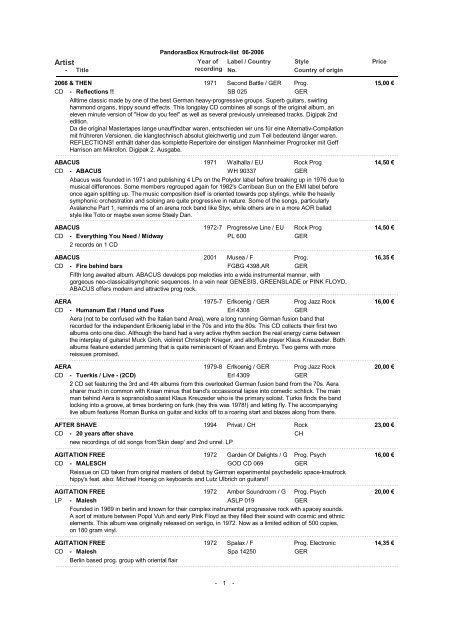The image depicts a black and white catalog listing various compact discs from different artists, primarily starting with the letter "A." Organized like a phone book, the artist names are aligned alphabetically down the left side, while columns across the top categorize the content by artist, title, year of recording, label, country/region, style, and price. The catalog seems to date back to June 2006 and features recordings primarily from the early 1970s, around 1971 or 1972. Most prices are listed in British pounds and range approximately from 14.50 to 16.35. Featured prominently are multiple entries from the artist Abacus with albums like "Reflections" and others, as well as other artists like Aftershave and Agitation Free. The text throughout the document is fine and somewhat challenging to read, with details becoming even more difficult to discern towards the bottom, which might indicate this is the first page of a larger collection.